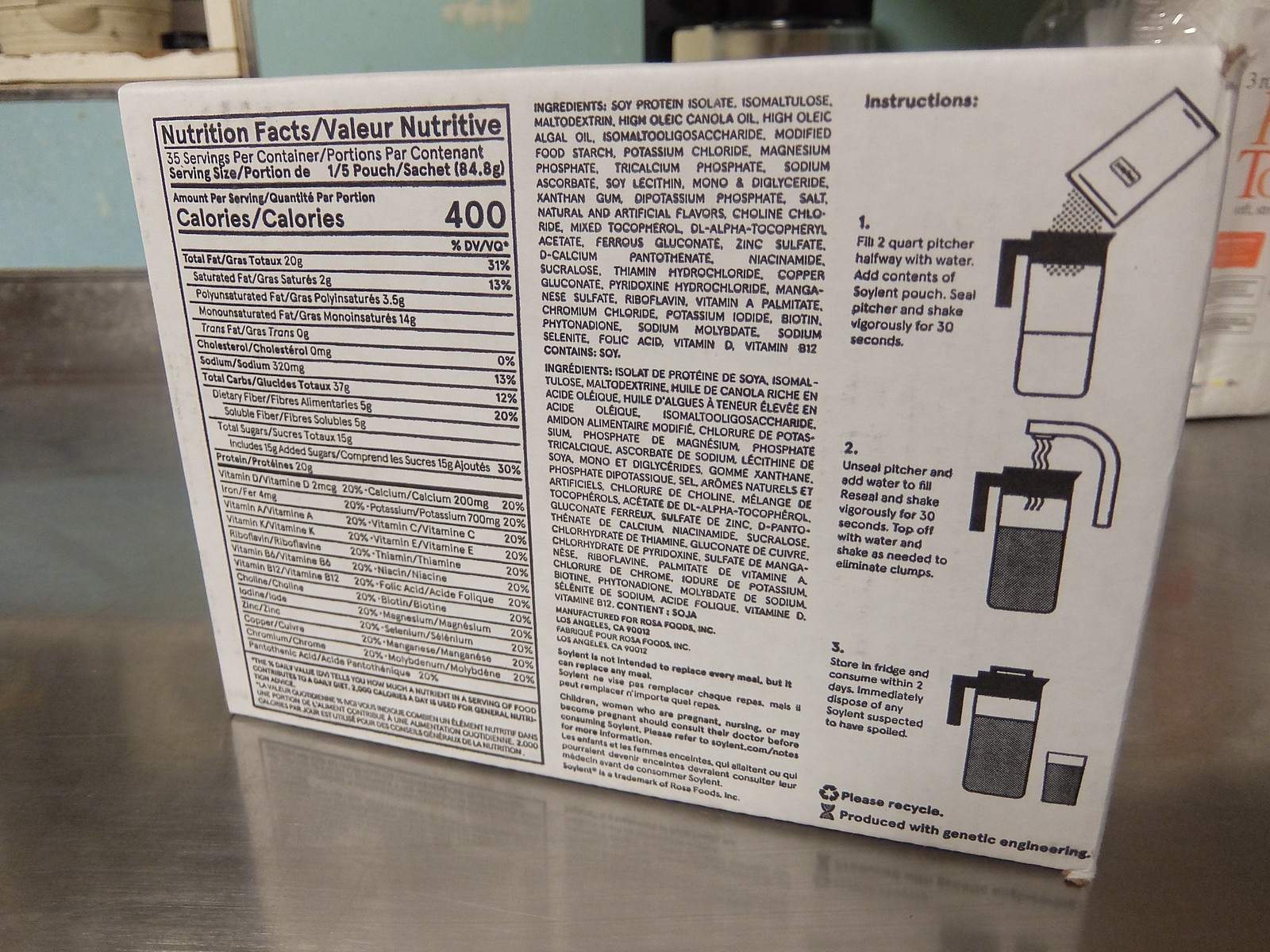The photograph features the back of a Soylent box, showcasing a detailed list of nutritional information and preparation instructions. The box contains 35 servings, with each serving providing 400 calories. The information is presented in multiple languages, catering to a diverse audience.

The instructions for preparing Soylent are as follows: 

1. Fill a two-quart pitcher halfway with water.
2. Add the contents of the Soylent pouch to the pitcher.
3. Seal the pitcher and shake vigorously for 30 seconds.
4. Unseal the pitcher and add more water until it is full.
5. Reseal and shake again for 30 seconds.
6. Top off with additional water if necessary and shake as needed to eliminate clumps.
7. Store the pitcher in the refrigerator and consume the prepared Soylent within two days.
8. Immediately dispose of any Soylent that is suspected to have spoiled.

The packaging is labeled “Soylent,” produced by Rosa Foods based in Los Angeles, California. It provides a comprehensive list of ingredients and nutritional facts, emphasizing the product's purpose and preparation method.